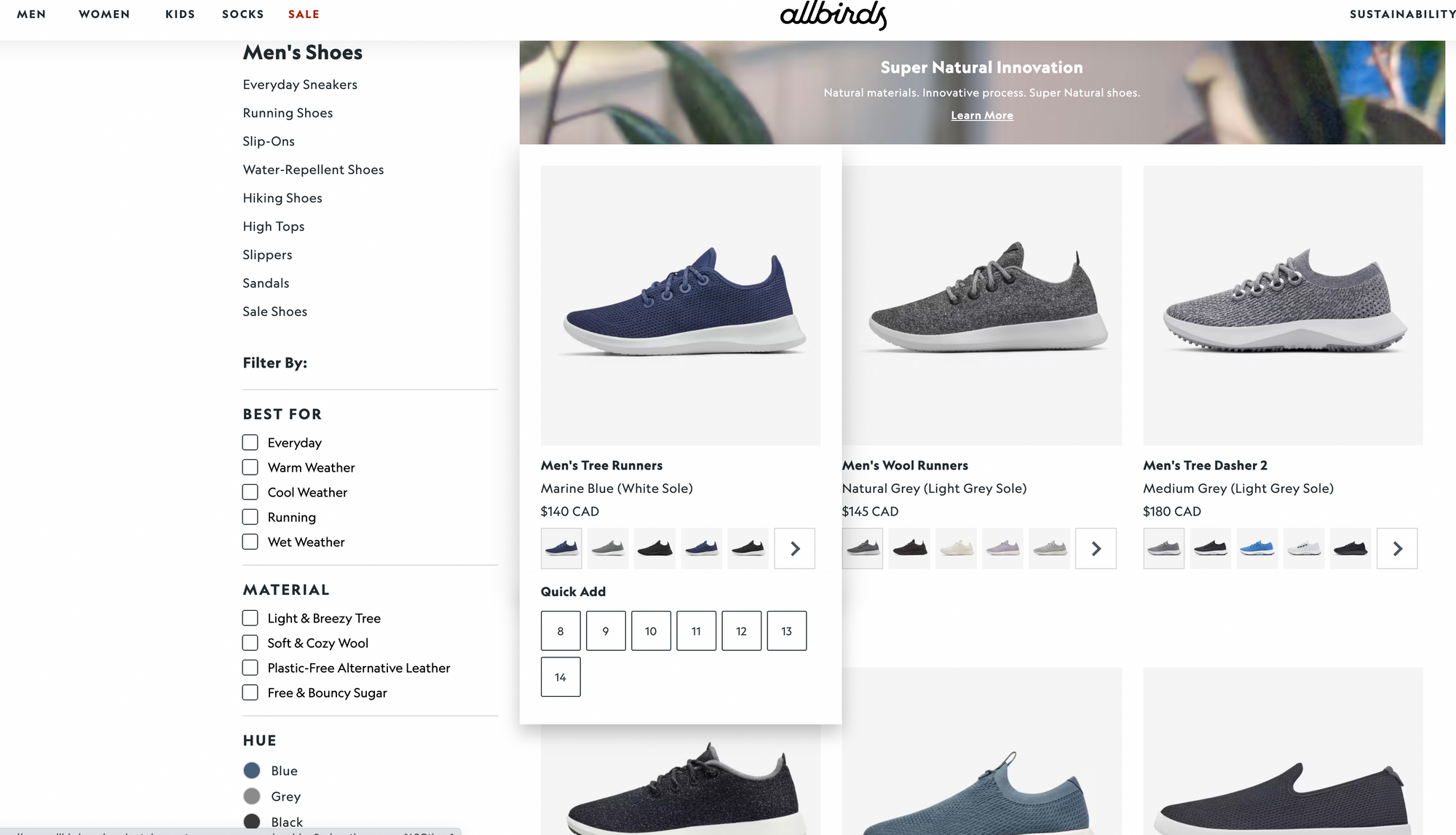**Caption:**

Allbirds Shopping Website Interface

The Allbirds shopping website offers a detailed and user-friendly interface for purchasing their highly acclaimed wool sneakers. The top menu features categories for Men, Women, Kids, Socks, and Sale items. Notably, the Sale category is highlighted in red, while the others are listed in black for easy navigation.

The men's shoes section is prominently displayed, showcasing various types of footwear including everyday sneakers, running shoes, slip-ons, water-repellent shoes, hiking boots, high-top slippers, sandals, and sale items. Users can refine their search with filters categorized as best suited for everyday use, warm weather, cool weather, running, and wet weather.

Material options are described as light and breezy, soft and cozy, plastic-free, and sugar-based, promoting the brand's commitment to sustainability. Color options such as blue, gray, and black are available, each represented by a corresponding color circle for quick selection.

To the right of the filters, images of the sneakers provide a clear view of the products. Above the product images, the phrase "Supernatural Innovation" is prominently displayed, highlighting Allbirds' innovative approach to footwear design. Users can click on the images to check the availability of sizes. However, the display is limited to showing only six sneakers at a time.